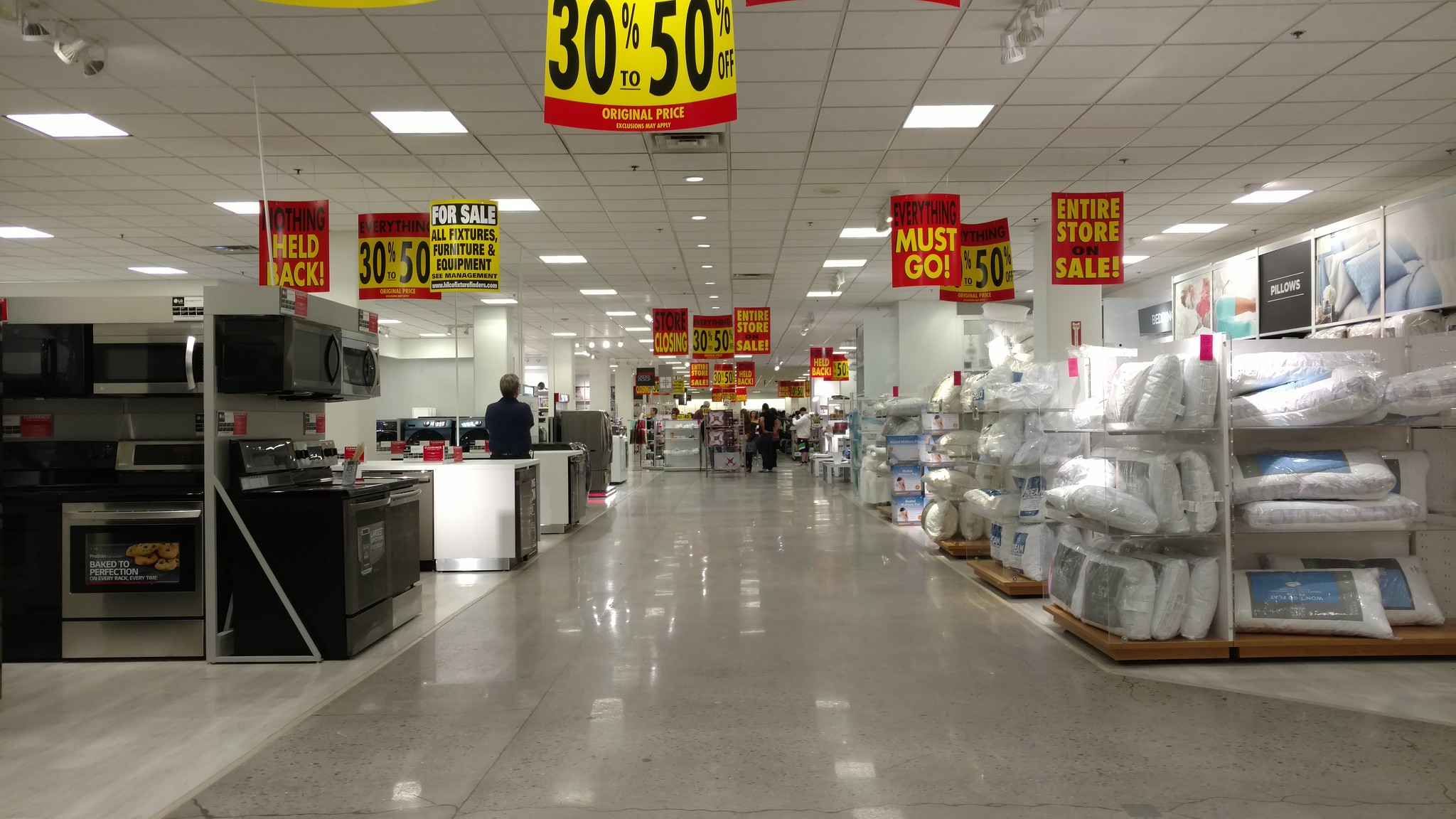This photograph depicts a bustling aisle in a department store. The perspective is from the middle of a hallway, revealing a ceiling adorned with white tiles from which several signs hang. Foremost among these is a prominent yellow sign with a red base, proclaiming "30 to 50% off." To the left, an assortment of appliances is displayed, including stovetops and microwaves. Further down this aisle, a man stands with his back to the camera, appearing to examine a section that likely contains washers and dryers. On the upper right side of the image, rows of pillows are neatly arranged under another eye-catching red sign that declares "Entire store on sale. Everything must go." The scene encapsulates the vibrant and busy nature of a retail environment amidst a significant sale event.